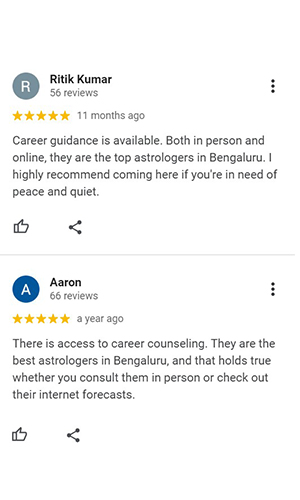This image appears to be a screenshot of a review section, showcasing feedback from two different users about a service related to astrology and career guidance in Bengaluru.

The first review is by Riddick Kumar, whose profile image is represented by the letter "R" inside a greenish-gray circle. Kumar's review count stands at 56, and he has given a full 5-star rating. His review, posted 11 months ago, reads: "Career guidance is available both in person and online. They are the top astrologers in Bengaluru. I highly recommend coming here if you are in need of peace and quiet."

Below Riddick's review is another one by a user named Aaron, identified by a profile picture with the letter "A." Aaron, who posted his 5-star review a year ago, writes: "There is access to career counseling. They are the best astrologers in Bengaluru, and that holds true whether you consult them in person or check out their internet forecast."

Each review has interactive icons for a thumbs up and sharing, allowing other users to engage with the feedback.